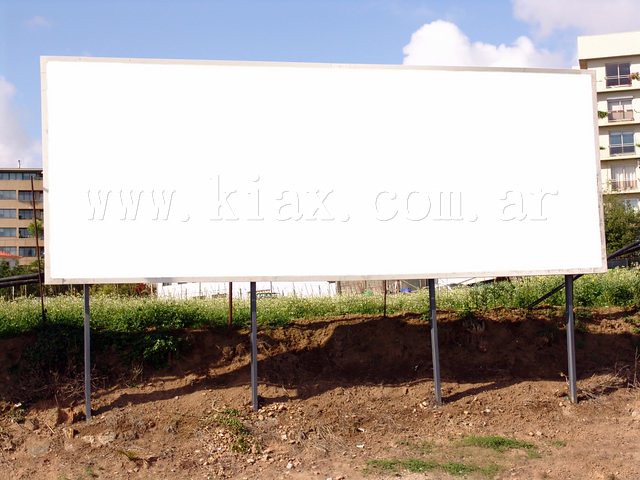The photograph captures a large, rectangular white billboard mounted on four metal posts, contrasting against a bright blue sky with scattered white clouds. The billboard, outlined in beige, prominently displays the web address www.kiax.com.ar. The structure is anchored in a patch of brown dirt, with scattered green grasses around its base. Surrounding the billboard, the scene includes several buildings: a white apartment building with balconies and at least five floors to the right, and a four-story brown building with numerous windows and an awning to the left. A smaller white building appears faintly in between. The overall setting suggests an urban area with a mix of residential architecture and open grounds.